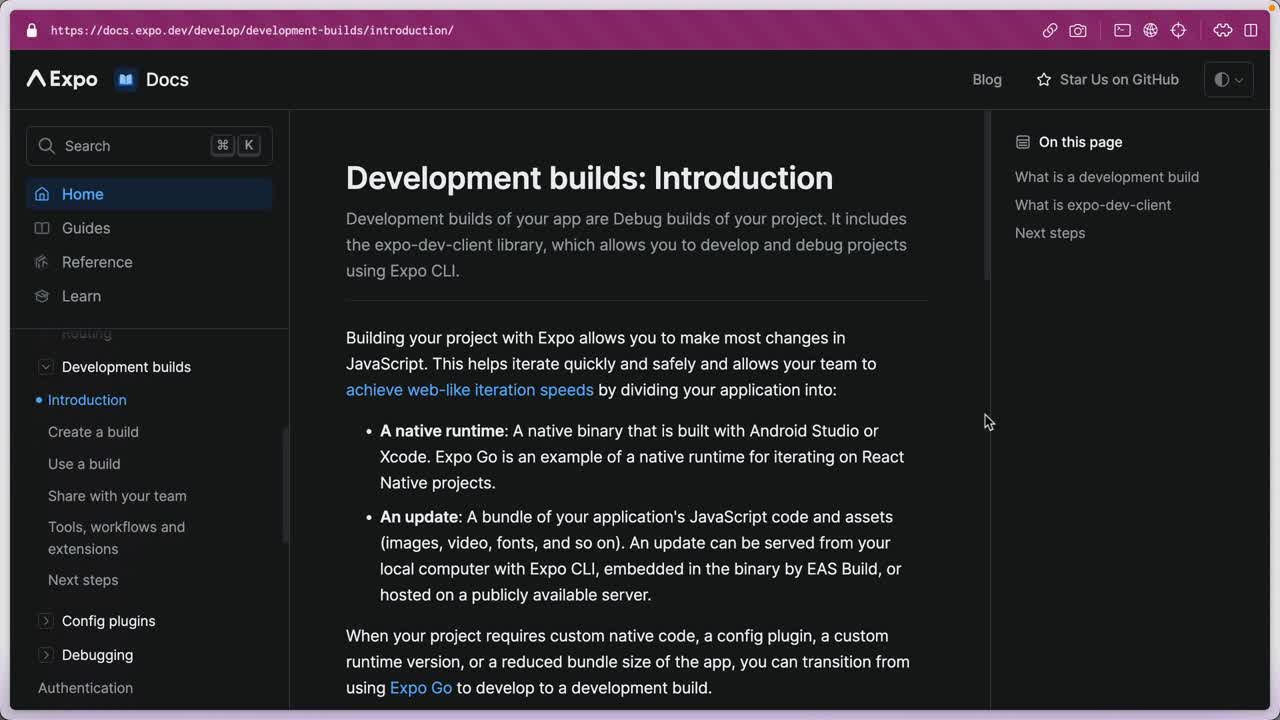The image captures a web page with a predominantly black background and white text. At the top left corner, the page header displays "Expo" followed by "Docs" to the right. Adjacent to this, on the right side of the top bar, which is purple, there are options such as "Blog" and "Star us on GitHub." On the left, running down the side, is a navigation menu featuring options like Home, Guides, Reference, Learn, Development Builds, Introduction, Create a Build, Use a Build, and a search bar.

The central focus of the page is the main content section, prominently displaying the titles "Development Builds" and "Introduction." The text explains that development builds of an app are debug builds, including the Expo Dev Client Library, which aids in developing and debugging projects using the Expo CLI. The content elaborates on how building projects with Expo permits rapid and safe iteration by making changes primarily in JavaScript, allowing teams to achieve web-like iteration speeds through the division of the application into two bullet-pointed sections.

At the bottom of the page, it is mentioned that if a project requires custom native code, a config plugin, a custom runtime version, or a reduced bundle size, one can transition from using "Expo Go" to a development build. Some of the significant phrases such as "achieve web-like iteration speeds" and "Expo Go" are highlighted in blue.